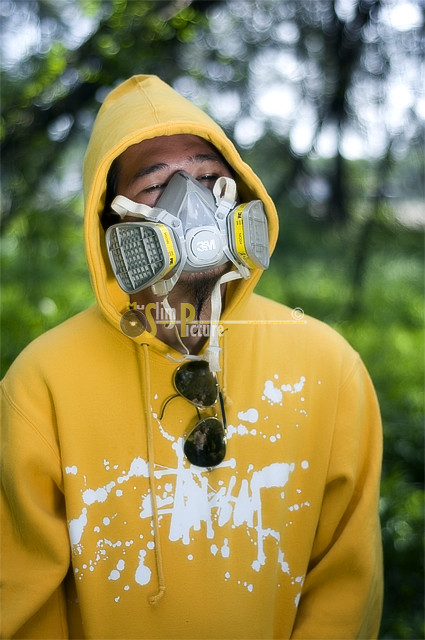In the image, we see a man wearing a silver gas mask prominently featuring the 3M brand in white, with two filters on either side and white straps securing it to his face. He is facing the camera with his eyes closed. He is dressed in a vivid yellow hoodie adorned with a splotchy white graphic on the front, which resembles random paint splatters but might be a stylized print or tagger's signature. The hoodie covers his head, and a pair of sunglasses is tucked into the bottom of the hood. The background is blurred with a bokeh effect, showcasing a natural setting with the trunks of trees and greenery, and hints of blue light likely filtering through as the sky. The scene suggests that the man might be a graffiti artist or involved in some artistic endeavor outdoors.